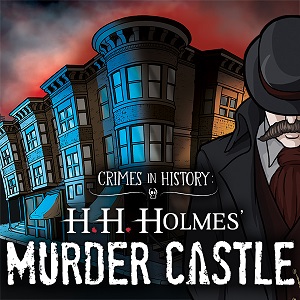The image is a small, pixelated, square illustration, measuring about 2 inches by 2 inches, resembling an app icon or YouTube thumbnail. It features a color cartoon depiction of a corner section of traditional European-style row houses, possibly hinting at Baker Street from the Sherlock Holmes series. Above the stone buildings, the sky transitions from a vibrant red to dark gray clouds. On the right side of the image, a man with light skin, a long handlebar mustache, and a tilted black bowler hat and jacket is visible, though his eyes are not shown and his face is partially cropped. In the center of the illustration is white text that reads "Crimes in History," accompanied by a small skull graphic with radiating lines. Below this, in bold white stencil font, it says "H.H. Holmes," with red periods between the initials, and just beneath, "Murder Castle." The overall style blends color illustration with prominent textual elements.